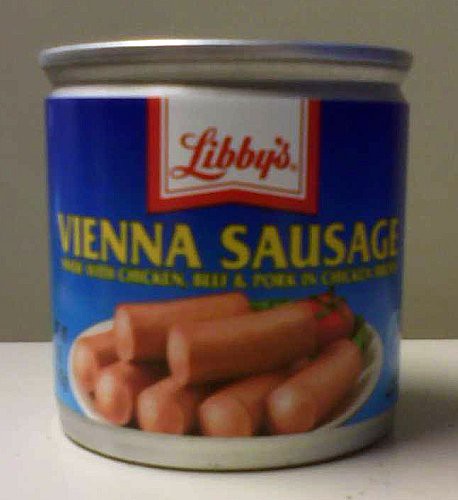The image features a close-up shot of a small can of Vienna Sausage by the brand Libby's. The can is silver and cylindrical, with the label transitioning from a dark blue at the top to a lighter blue at the bottom. The Libby's logo appears prominently at the top center of the label; it is designed in a white script set against a red and white ribbon-like emblem. Below the logo, in bold yellow text, are the words "Vienna Sausage," and additional text describing the contents as a blend of chicken, beef, and pork, though the details are somewhat blurred. An image on the label displays a serving suggestion, featuring a plate with seven light brown, smooth-textured, cylindrical sausages arranged neatly, accompanied by a tomato. The can rests on a white table, with an olive green-colored wall in the background, creating a subtle contrast.